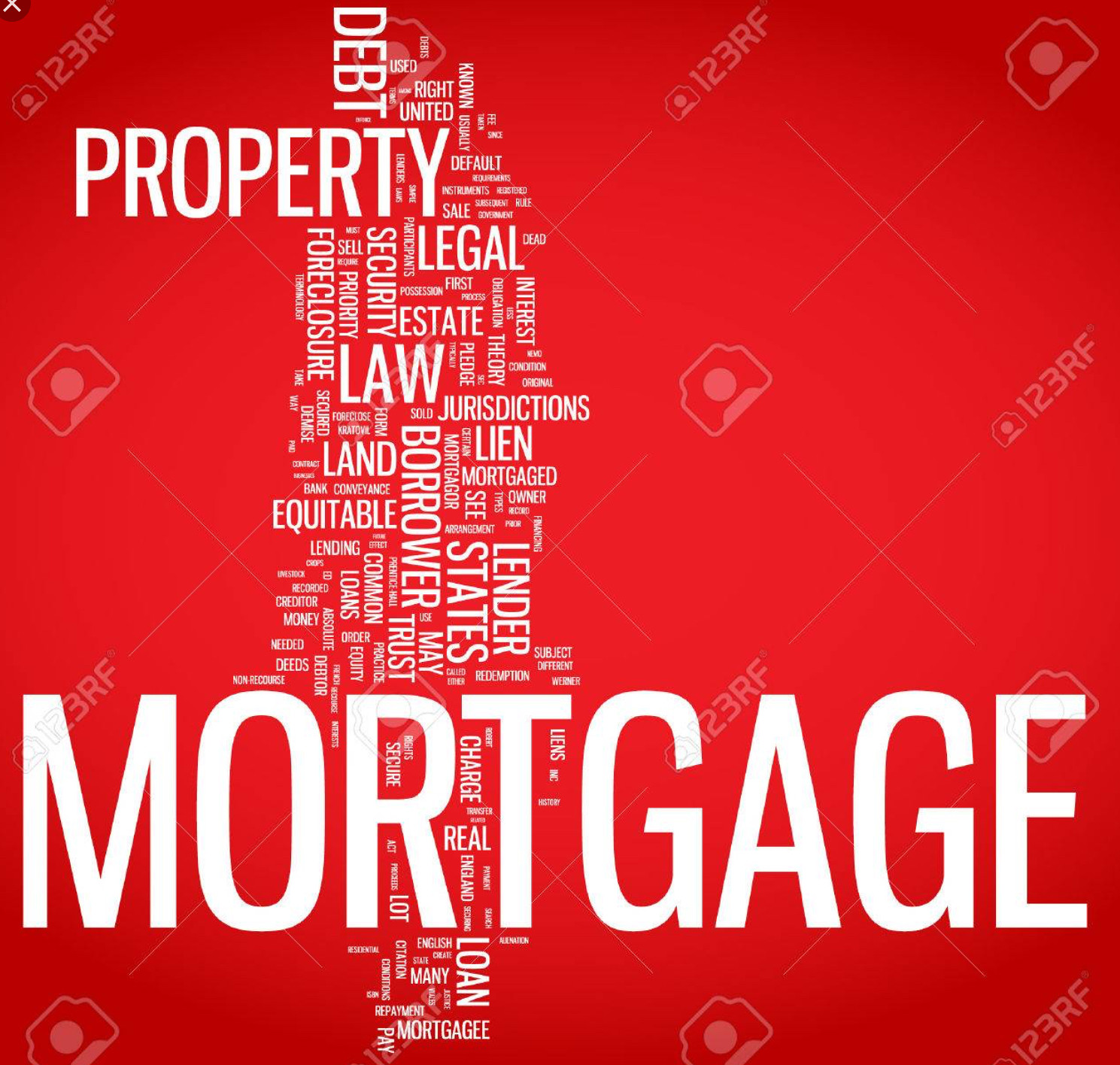The image is a vibrant red poster featuring a variety of white capitalized words associated with property and finance. Prominently placed near the bottom, the word "MORTGAGE" stands out in large letters. Vertically aligned near the middle of the image is the word "DEBT," while "PROPERTY" is written horizontally. Other significant terms such as "LEGAL," "FORECLOSURE," "SECURITY," "LAW," "LOAN," "BORROWER," and "LENDER" are scattered across the poster, both horizontally and vertically. Additional words like "ESTATE," "LIEN," "JURISDICTION," "COMMON," "EQUITABLE," "REAL," "RIGHT," "UNITED," "DEFAULT," "TRUST," and "STATES" create a textual pattern forming a stripe down the first third of the poster. The design also includes smaller, harder-to-read text and has cartoon-like figures, with stock image symbols subtly incorporated into the background.